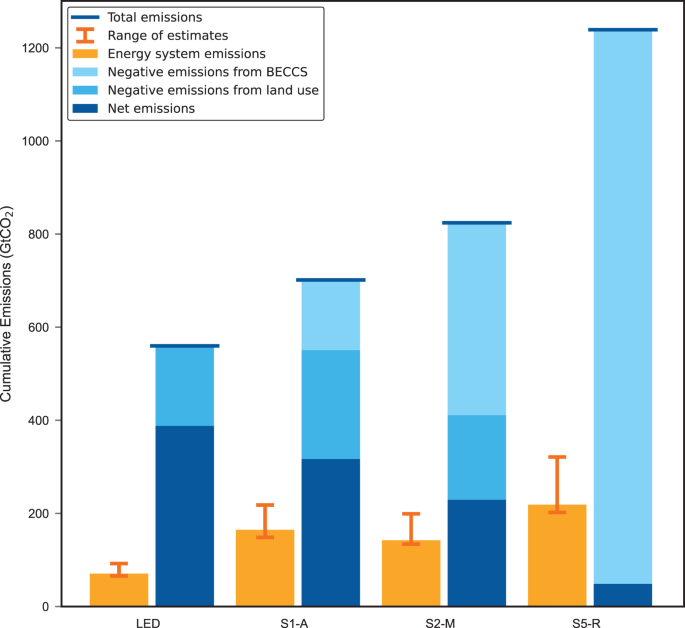The image depicts a detailed bar graph with a white background, illustrating cumulative emissions in gigatons of CO2 (GTCO2) on the y-axis, ranging from zero to 1,200, and various categories on the x-axis labeled LED, S1-A, S2-M, and S5-R. Each category contains two bars: an orange bar representing energy system emissions and a stacked bar in differing shades of blue. These blue bars display total emissions, negative emissions from BECCS (Bioenergy with Carbon Capture and Storage), negative emissions from land use, and net emissions. Accompanying the graph is a legend in the top left corner, detailing the colors and corresponding categories. The graph is ordered with the largest emissions bars on the right and the smallest on the left, indicating emissions associated with four different technologies or scenarios. Additionally, a bold capital "I" on the graph indicates a range of estimates, highlighting variability in the data.